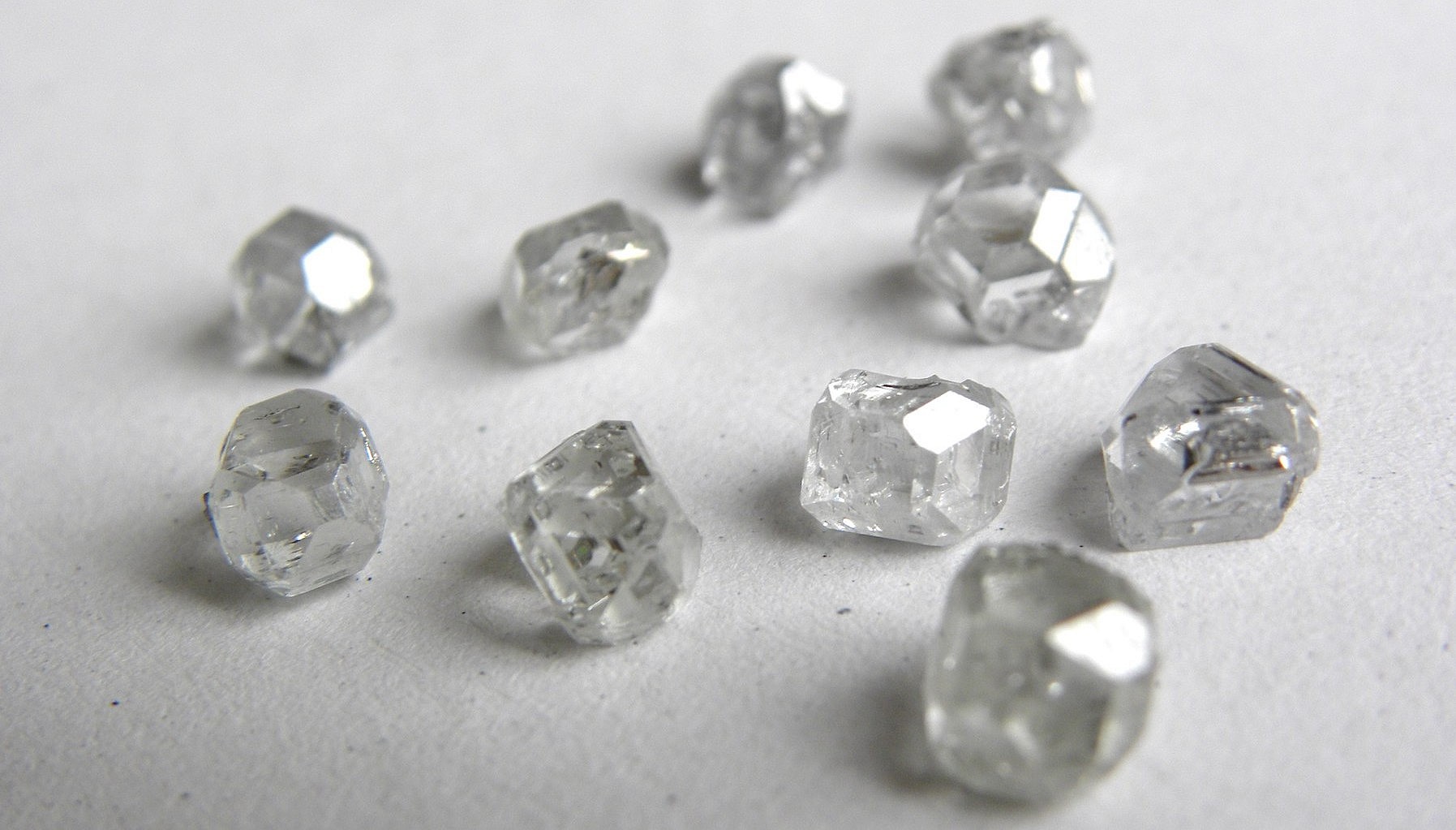The image features a collection of 10 distinct gemstones displayed on a rough, predominantly white surface that includes scattered black specks. The gemstones exhibit a range of geometric shapes, with some being circular while others have more squared-off appearances, yet all possess flat facets that contribute to their symmetrical forms. Although not highly polished, these crystal-like objects resemble diamonds or similar gems and showcase colors primarily in shades of gray, white, black, and a clear, translucent hue.

The arrangement of the gemstones creates a visually intriguing pattern. On the left half of the image, four stones form a near-perfect square. The remaining six stones are arranged into two different triangular formations: the lower triangle points downward, while the upper triangle, positioned above and at roughly the two o’clock direction relative to the lower one, points outward.

Occupying most of the image, the placement of the gemstones centers them in the frame, leaving little empty space and highlighting their intricate details. This composition could easily be featured on a jewelry website or as part of a stone collector's display.